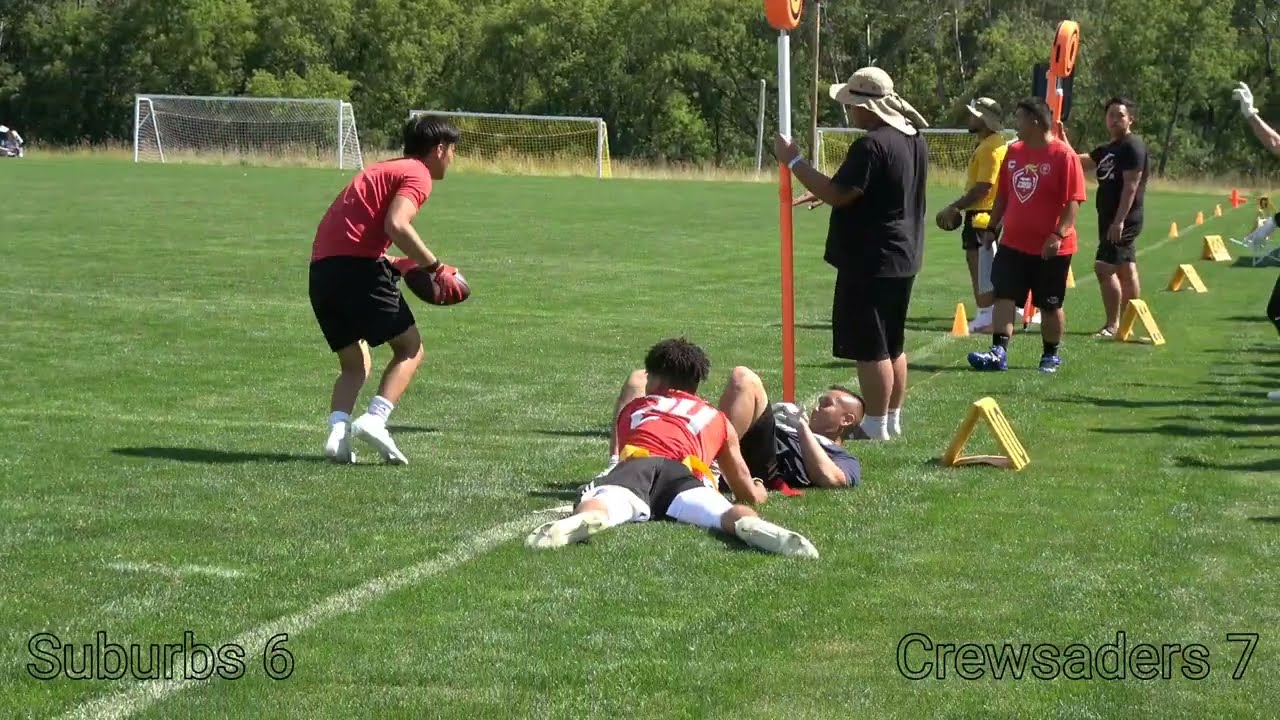The photograph captures an energetic moment during a practice session on a green rugby or football field, predominantly featuring Asian players. The lush grassy field stretches out with white boundary markers and yellow placement lines. Central to the image, a player dressed in a red t-shirt, black shorts, white shoes, and red gloves is seen in motion, holding a football and running up the field with his back turned to the camera. The field is dotted with three soccer nets positioned in the distance. 

To the left of the frame and bisected diagonally by a white line, two individuals in black t-shirts and shorts are visible, holding orange first down markers, signaling the locations for first and second downs. These markers help delineate the field's functional zones. Adjacent to them, nearer the center of the frame, two players are seen resting on the ground, one in a red jersey and the other in a yellow jersey. One lies on his back, and the other on his stomach, both seemingly observing the action on the field.

The backdrop of the image includes a small, verdant forest, adding a natural boundary to the scene. Notably, the photograph is watermarked at the bottom: "Suburb 6" on the left and "Crusaders 7" on the right, both in a transparent font with a black border. This caption lends a sense of authenticity to what appears to be a dynamic training or friendly match involving the Crusaders team.